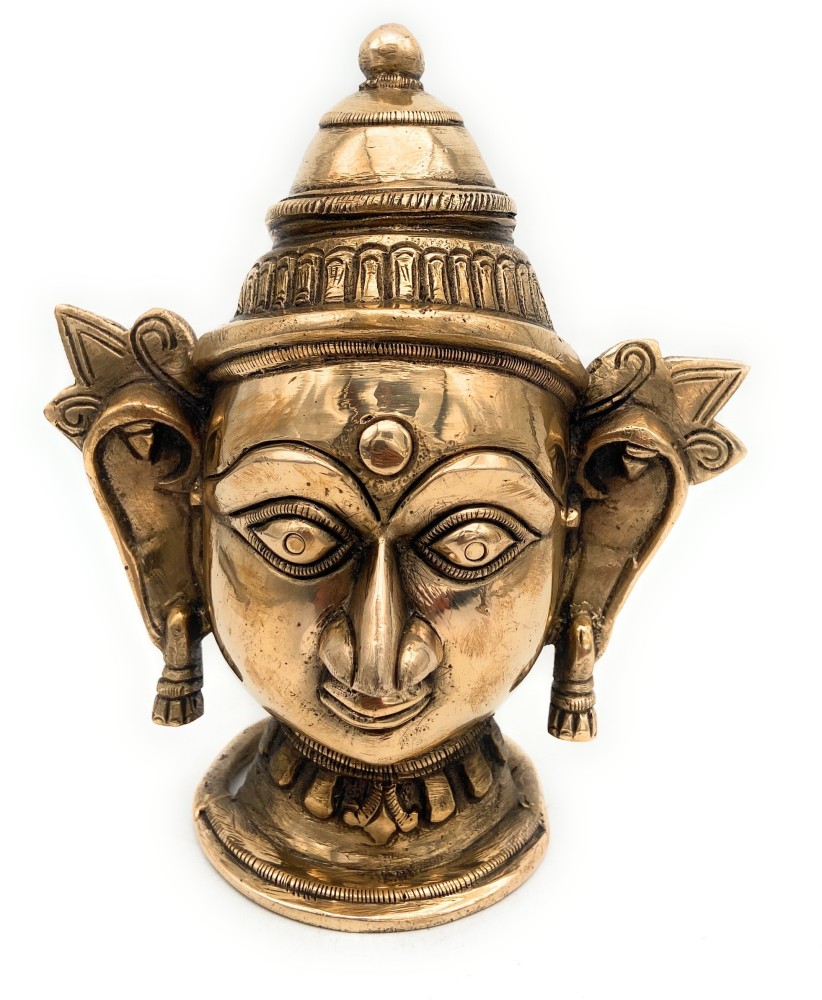This image features a detailed gold metallic bust of a deity, possibly of Hindu origin, though some elements suggest Egyptian influence. The headpiece includes a hat adorned with repetitive etched details, including rows of rectangles and a band running around its circumference, culminating in a small ball at the top. The face exhibits a rounded chin and cheeks, with prominent, wide eyes that possess segmented tube-like details around them. The pupils are inset from the same material. A large circular dot is positioned in the center of the forehead. The statue's nose is pronounced, situated above small lips. Large ears, with spiked triangular adornments at the top, hold tassel-style dangling earrings. The neck is encircled by a necklace featuring a segmented band design, from which five flaps hang down. The base of the bust is shiny, complemented by a small segmented coil on its front half. There are intricate carvings circling the very base of the statue, which stands out against the plain background.